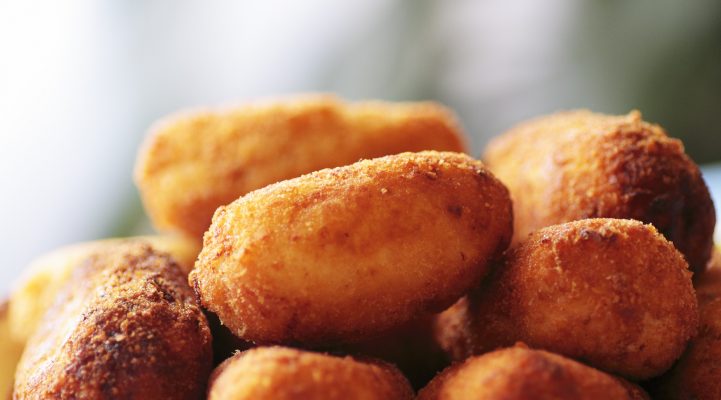The image showcases a close-up of a pile of deep-fried nuggets with a crispy brown exterior, varying in shades from golden to dark brown. The nuggets, which could be made of cheese, meat, or vegetables, have a rounded, oval shape reminiscent of chicken nuggets or mini cocktail franks. There are approximately eight pieces visible, with some stacked on top of each other. The photo's depth of field focuses on the nuggets in the foreground, highlighting their crisp, unseasoned breading. The background is blurred, displaying a mix of white and green colors, which contrasts with the detailed textures of the fried food. One nugget, located in the bottom left corner, appears slightly burnt, adding to the range of brown hues in the image. The close-up nature of the photograph captures the savory appeal and crunchy texture of the deep-fried treats.